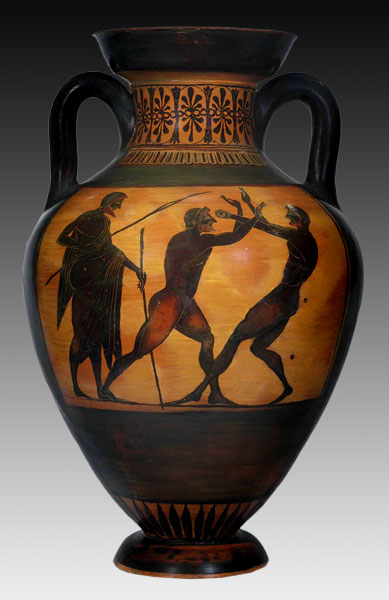This photograph captures an ancient Grecian urn with a rich and intricate design. The urn features two symmetrical handles that extend from the neck to the body, both painted in solid black. The vase itself is predominantly black, with decorative segments highlighting antique artistry. At the neck, there's an intricate floral pattern in black against an orange background, accentuating its classical elegance.

Below the floral motif, the urn's body showcases a dynamic combat scene. The scene, set against a gold background, depicts three men deeply engrossed in fierce hand-to-hand combat. The man on the left, possibly clad in a robe or holding one, is an observer, gripping two spears and poised for action. The central figure, characterized by exceptionally muscular, powerful thighs and adorned in what appears to be minimal clothing, engages with an opponent to his right. His forward-straining posture—with brawny arms outstretched—conveys the intensity of the struggle. Meanwhile, his adversary to the right, possibly wearing a headband or blindfold, leans back defensively, one leg bent and the other extended straight down.

The lower part of the urn features a thick black band beneath the combat illustration, succeeded by another sequence of black stripes on an orange field, before merging into the solid black base. The meticulous details of the figures—though sometimes exaggerated—alongside the carefully crafted decorative elements, vividly evoke the craftsmanship and thematic preferences of ancient Greek art.